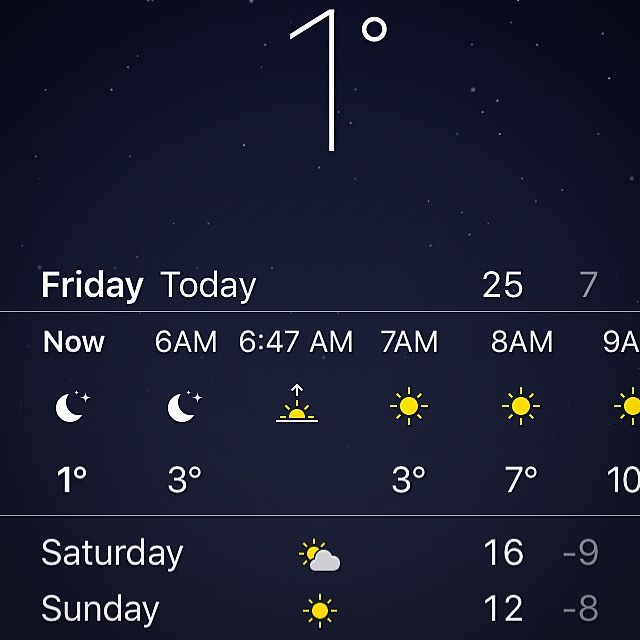A screen print, likely taken from a cell phone or computer, displays weather information against a black background. At the top, in large white font, it reads "1°". The line below, in smaller white font, states "Friday, today 25°" with a low of "7°" rendered in gray. Following this, the next section begins with "Now" in white font. Adjacent to this text, there's a moon icon accompanied by stars, indicating "1°". 

Beneath this, it lists "6 a.m." with another moon icon and the temperature "3°". At "6:47 a.m.", a sunrise symbol appears. By "7 a.m.", a yellow sun icon is displayed, showing "3°". Continuing, "8 a.m." is marked with another yellow sun icon and the temperature "7°". 

At "9 a.m.", although the 'M' in 'a.m.' is truncated and the sun icon is mostly visible, it signifies a temperature of "10°" with part of the degree symbol cut off. 

Towards the bottom, the weather forecast for "Saturday" is presented in white font with a cloudy icon. The high temperature is indicated as "16°" and the low as "−9°", the latter in gray font. Below that, "Sunday" appears in white font, flanked by a sun icon. The high is "12°" and the low is "−8°".